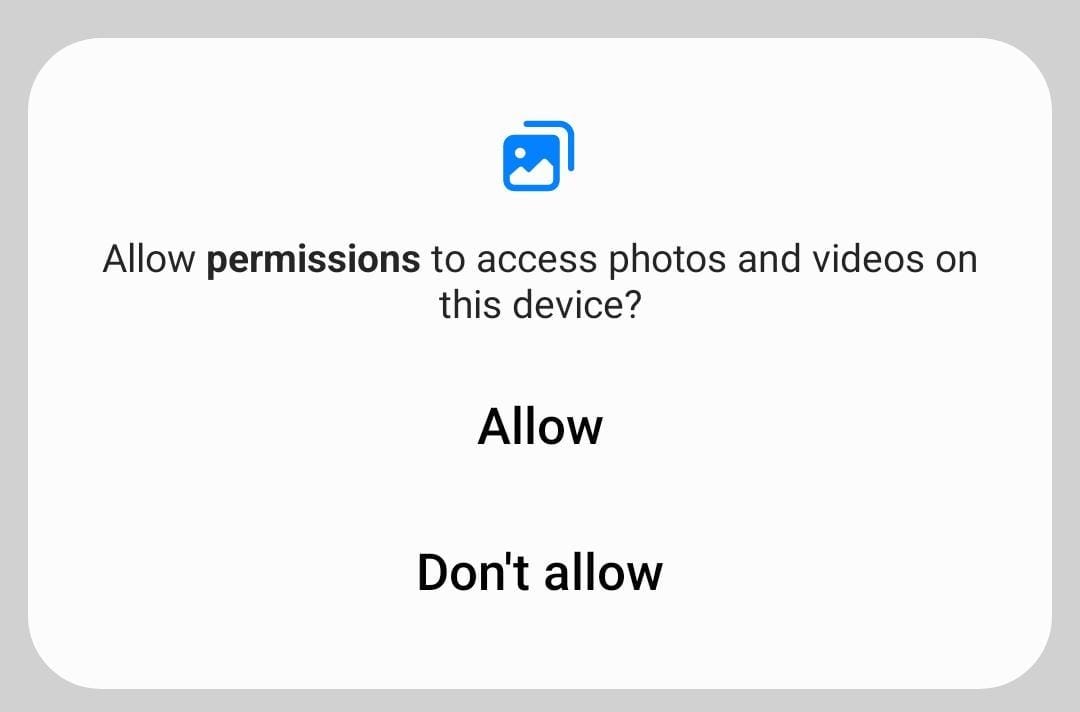The image features a notification popup set against a grayish, square background. The popup itself has a white background and is centrally located within the image. At the center of the popup is a blue square containing a white dot, along with two curved lines that resemble a rooftop. Above this icon is an upside-down L-shaped line. 

The notification text is displayed in black font with varying shades. The text reads: "Allow permissions to access photos and videos on this device?" The word "Allow" is in a bolder, darker font, while "permissions" returns to a lighter shade.

Below the text, prominently centered, is the word "Allow" in a larger, thicker font. Directly beneath this, there is an option stating "Don't Allow" in a rounded-edge square button with a white background, outlined by a gray border.

The popup box has a thicker gray border on all four edges, with the top edge being slightly thicker than the others. The bottom and side edges are thinner.